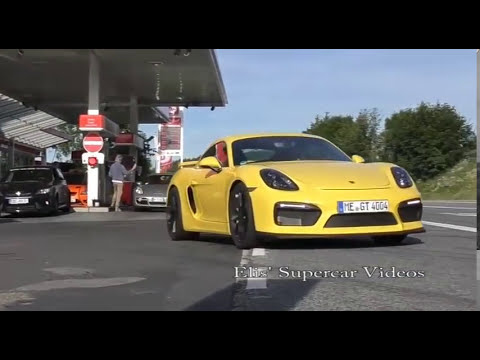The photograph, appearing to be a still from a video, captures a scene at a European gas station on a clear day. Dominating the foreground, a yellow Porsche 911 with a European license plate reading "MA GT4004" is parked slightly angled towards the road, its black-rimmed wheels catching the eye. Just behind it, at one of the red gas pumps under a tall flat roof, a man in a bluish jacket and brown khaki pants is reaching to fuel a gray Porsche, the same model as the yellow one. To the left, a lineup of additional vehicles, including an orange and a dark-colored car, are parked. The background reveals a small shop attached to the gas station, a gas price sign, trees, and a blue sky. In the bottom right corner of the image, white text reads "Eli's Supercar Videos," emphasizing the screenshot's origin from a video focusing on luxury vehicles.